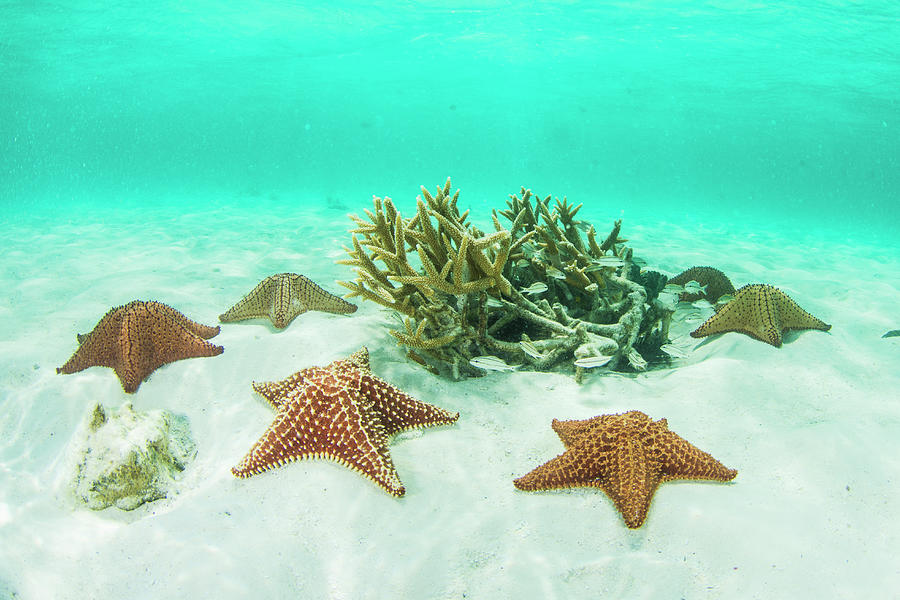The second image in the sequence is an underwater scene depicting vibrant marine life in shallow ocean water with a light blue tint. Central to the image is a coral reef showcasing a variety of colors, predominantly green and light brown, with its tree-branch-like formations adorned with spikes. Surrounding the coral, several starfish lay scattered atop the white sandy ocean floor. These starfish exhibit a range of colors and patterns, from reddish-brown with black spikes, to tans, maroons, and dark browns sporting lighter line patterns. The detailed marine tableau captures white and gray fish swimming near the coral, adding to the lively underwater environment. Around the reef, a conch shell lies on the sand, and a covered rock sits in the bottom-left corner, enhancing the scene's natural feel. Additionally, an unidentified black object extends from the right side of the frame, adding a touch of mystique to this captivating underwater landscape. The image provides a clear, shallow glimpse into oceanic life, showcasing vivid details and diverse sea creatures.